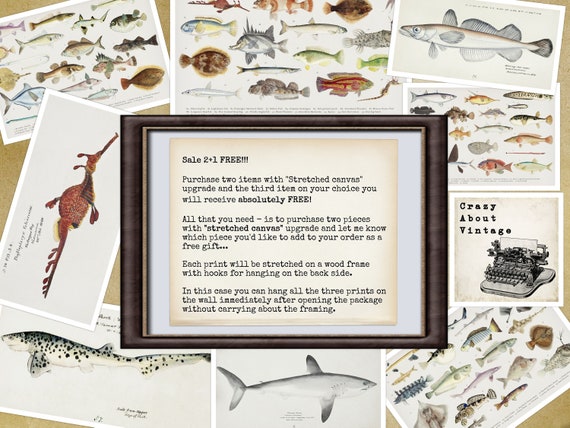The image depicts an array of nine detailed illustrations of various types of fish, potentially drawings or paintings, spread out on a surface that is mostly obscured but appears to be yellowish or tan. These illustrations encompass a diverse range of marine life, with some notable examples like a long, white and gray fish in the upper right corner. Central to the image is a dark brown wooden photo frame, containing a light brown paper with black text. The text, split into multiple paragraphs, includes a prominent message advertising a sale: "2 plus 1 free." It details a promotion where purchasing two items with a Stretched Canvas Upgrade grants a third item of your choice for free. The notice emphasizes that each print will be stretched on a wood frame with hooks for immediate wall hanging, eliminating the need for additional framing. Among the fish illustrations, there is also a notable poster featuring a typewriter with the phrase "crazy about vintage." The collection and arrangement suggest that these are examples of the items available for the promotional offer.